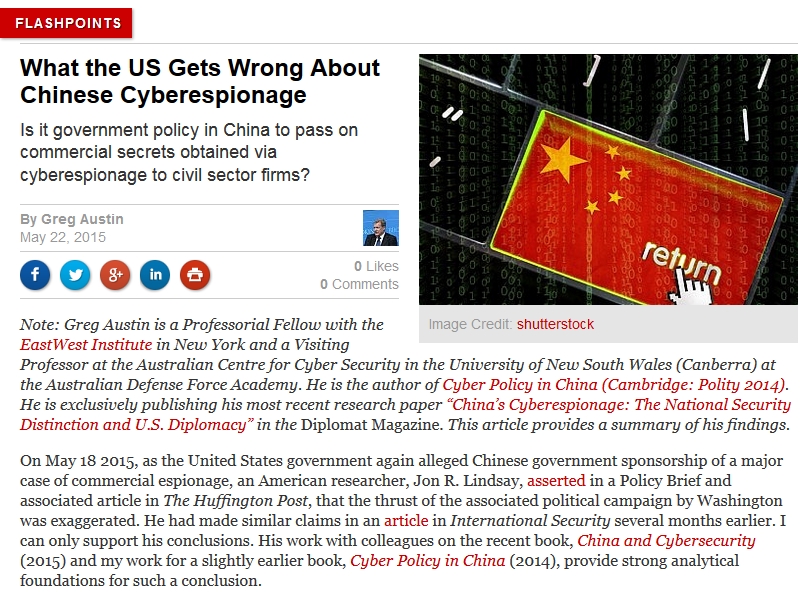The image is a screenshot from a website featuring an article. At the top of the screenshot, there's a small red banner with white text that reads "FLASHPOINTS" in capital letters. Below the banner, a thin line separates it from the main content area, which has a clean white background.

The article's title is prominently displayed: "What the U.S. Gets Wrong About Chinese Cyber Espionage?" Each major word is capitalized. Following the title, a subheading poses the question: "Is it government policy in China to pass on commercial secrets obtained via cyber espionage to civil sector firms?" 

Below this, the author, Greg Austin, is credited with a timestamp of May 22nd, 2015. Accompanying the article is a profile image of the author. Nearby, icons representing social media platforms are displayed, each showing zero likes and zero comments.

On the right side of the screenshot, adjacent to the author's name and the article title, there is an image of a keyboard. The section of the keyboard shown includes keys like the backslash and quotation marks. Notably, the "Return" key is highlighted in red with white text, and a small hand icon points to it. This key is styled with elements of the Chinese flag, featuring a large yellow star and four smaller stars.

The article content begins beneath these elements, continuing into the main body of the text.